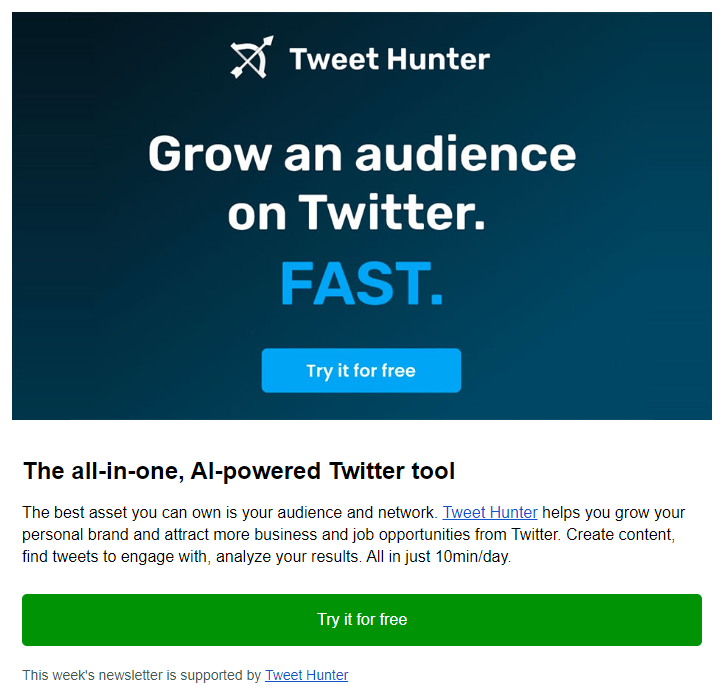Here is the cleaned-up and detailed caption:

---

The image features a promotional advertisement for TweetHunter on a blue background. At the top, the word "TweetHunter" is prominently displayed in white. Below it, there is a picture of a bow and arrow aimed towards the right. The image is accompanied by text that reads, "Grow an audience on Twitter, FAST." The word "FAST" is emphasized in all capital letters with a period at the end.

Underneath this main slogan is a blue clickable button labeled "Try for Free." Following the button, there is a bolded statement: "The all-in-one AI-powered Twitter tool."

The next section provides a detailed description of the service: "The best asset you can own is your audience and network. TweetHunter helps you grow your personal brand and attract more business job opportunities from Twitter. Create content, find tweets to engage with, and analyze your results—all in just ten minutes a day."

At the bottom of the image, there is another green button labeled "Try it for Free."

The final part of the image contains a note in blue, "This week's newsletter supported by TweetHunter," which is a hyperlink. Clicking it will take you directly to the TweetHunter website.

---